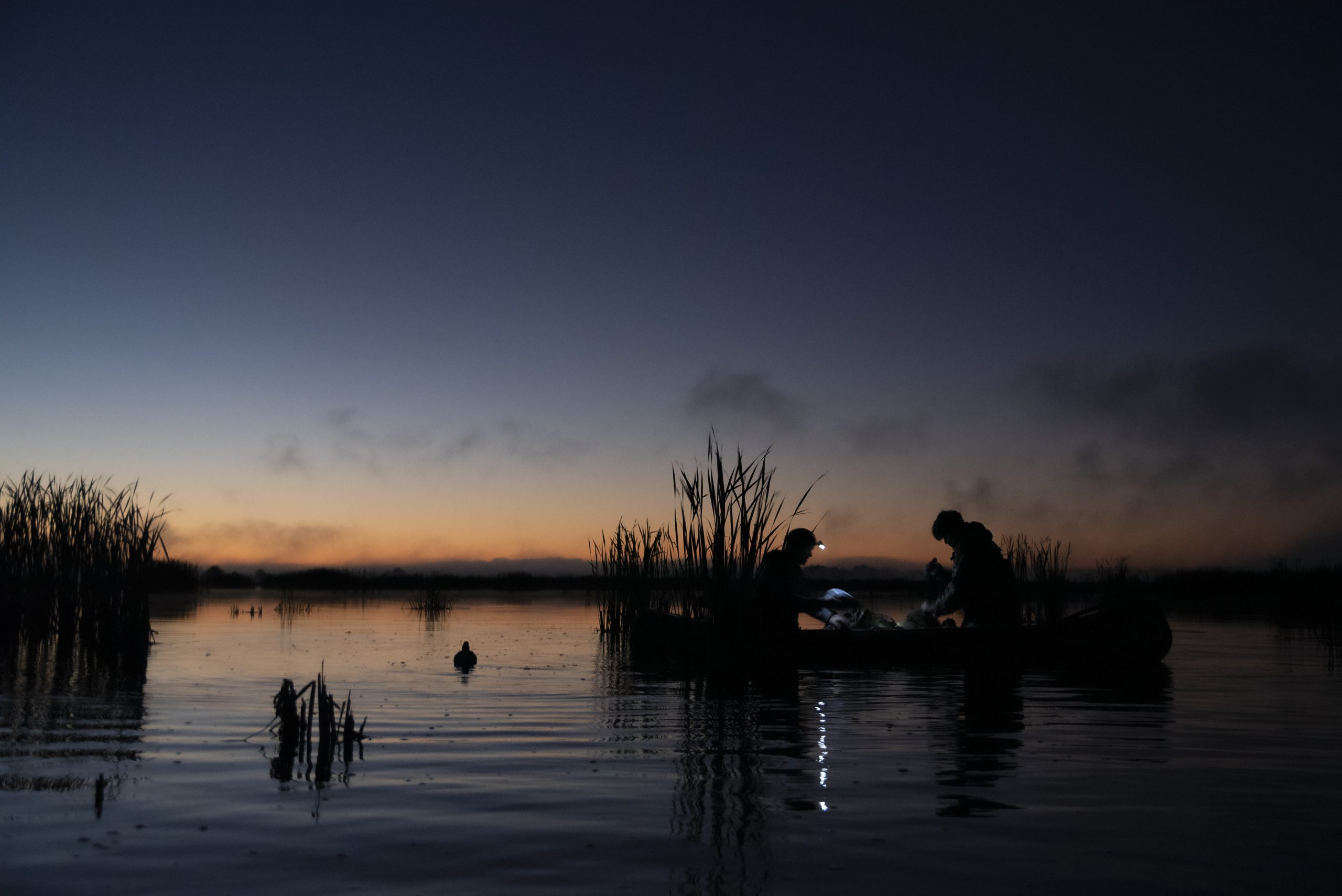At dusk or just before dawn, two fishermen are in a small boat situated on the right-hand side of a serene swamp. They're shining their lights into the boat, illuminating the calm water around them. The vibrant background features a stunning blend of dark sky and a gorgeous yellow and orange horizon, with scattered clouds adding texture. Surrounding their boat are various plants and stalks emerging from the water, both on the left and right, creating a harmonious natural setting. In the foreground to the left, additional stalks peek out just below the water’s surface. A duck or goose is visible between the boat and the left-side stalks, adding to the tranquil scene. Pieces of a wall can be seen in the distant background, hinting at nearby structures. One fisherman wears a light on his hat, while the other is hatless, and nestled between them appears to be a dog.